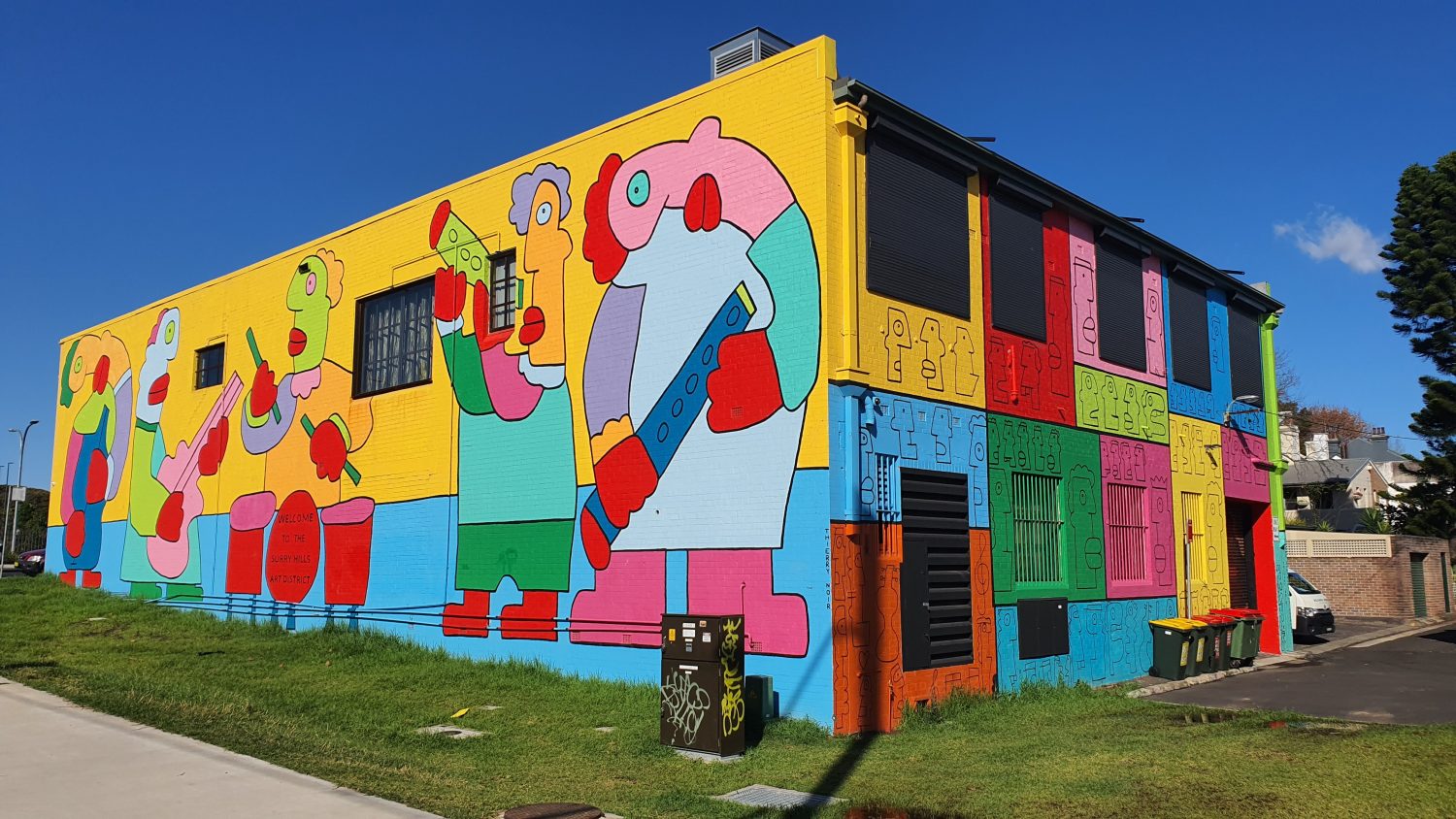In this vibrant and highly saturated photograph, a small brick building with a rectangular shape and flat roof stands as the focal point. The structure is adorned with colorful murals that dominate its facade. The side facing the right showcases a striking array of giant squares in vivid colors, each containing line-art faces resembling Maui Island heads. On the left side of the building, the murals shift to whimsical, Picasso-like abstracted figures with exaggerated, cartoonish proportions. These characters, painted in bright hues of pink, green, yellow, and blue, are depicted playing various musical instruments like flutes, drums, and guitars against a backdrop of yellow and blue. 

The surroundings add to the photo’s dynamic composition. The sky, edited to a surreal shade of bright blue, features a single cloud on this otherwise clear day. In front of the building, the grass appears green and lush but is more naturally grown rather than meticulously manicured. Additional elements like a bit of a car, a graffiti-tagged trash can, a section of road, and a tree partially visible on the right, blend seamlessly into the scene. Houses can be seen in the distance, completing the colorful, lively ambiance captured in this image.